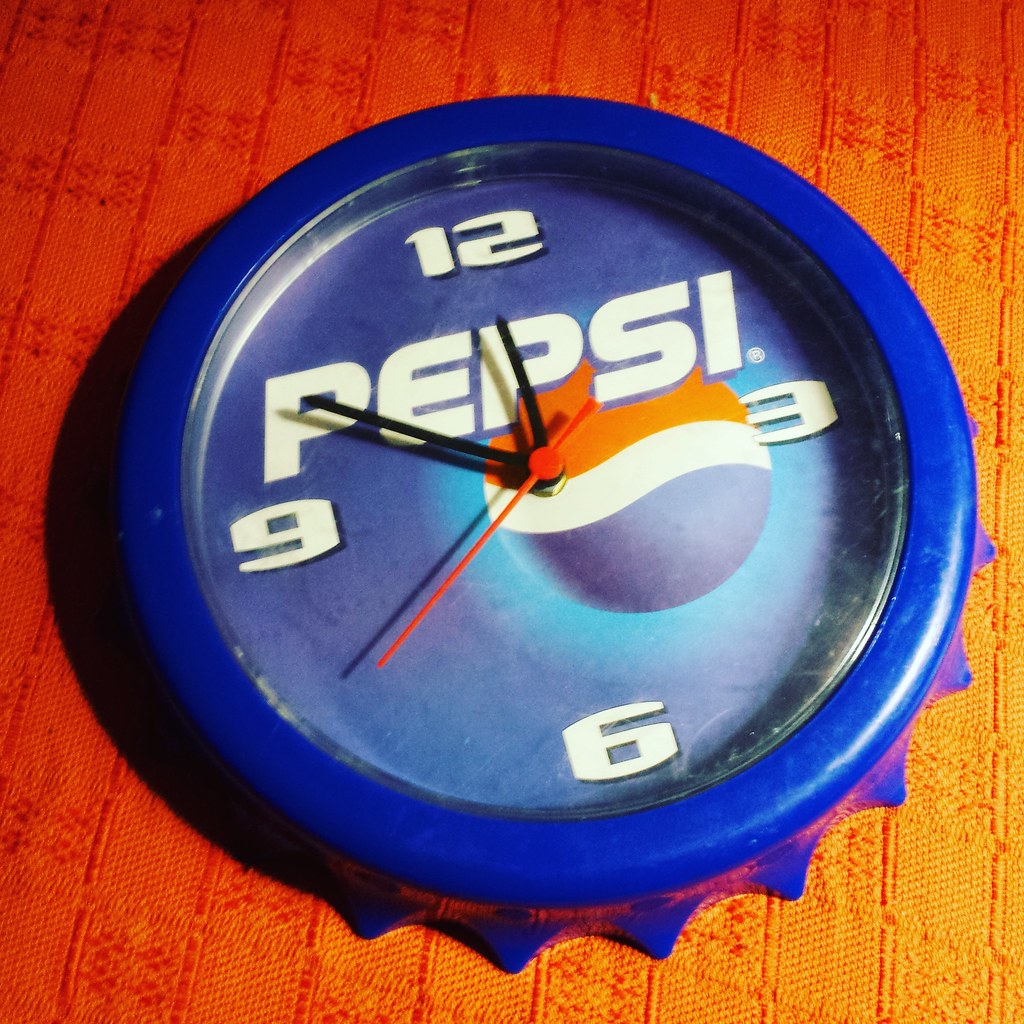This is a detailed photograph of a charming clock designed to resemble a Pepsi bottle cap. The clock's frame is colored in a deep blue and features serrated, pointy edges mimicking the cap of a bottle. This delightful wall clock prominently displays the Pepsi logo, which includes a circular design with red on the top, white in the middle, and blue at the bottom. The word "Pepsi" is emblazoned in bold white letters just below the number 12.

The clock face is divided into a blue outer ring and a lighter, almost turquoise inner section. Only the numbers 12, 3, 6, and 9 are marked, with the remaining positions left blank. The hands of the clock are black, while the second hand is a vivid red, and it reads approximately 11:50:40.

The clock appears to rest on a surface or wall against a background of an intricate, dark orange fabric that gradually transitions to a yellowish hue due to lighting. This fabric could potentially be a tablecloth, placemat, or carpet with tiny, detailed squares that add texture to the scene. The clock is slightly tilted with the 12 inclined toward the top left corner of the photograph, giving it a quirky and playful appearance. The overall aesthetic and whimsical design of the clock make it a particularly cute and eye-catching piece.